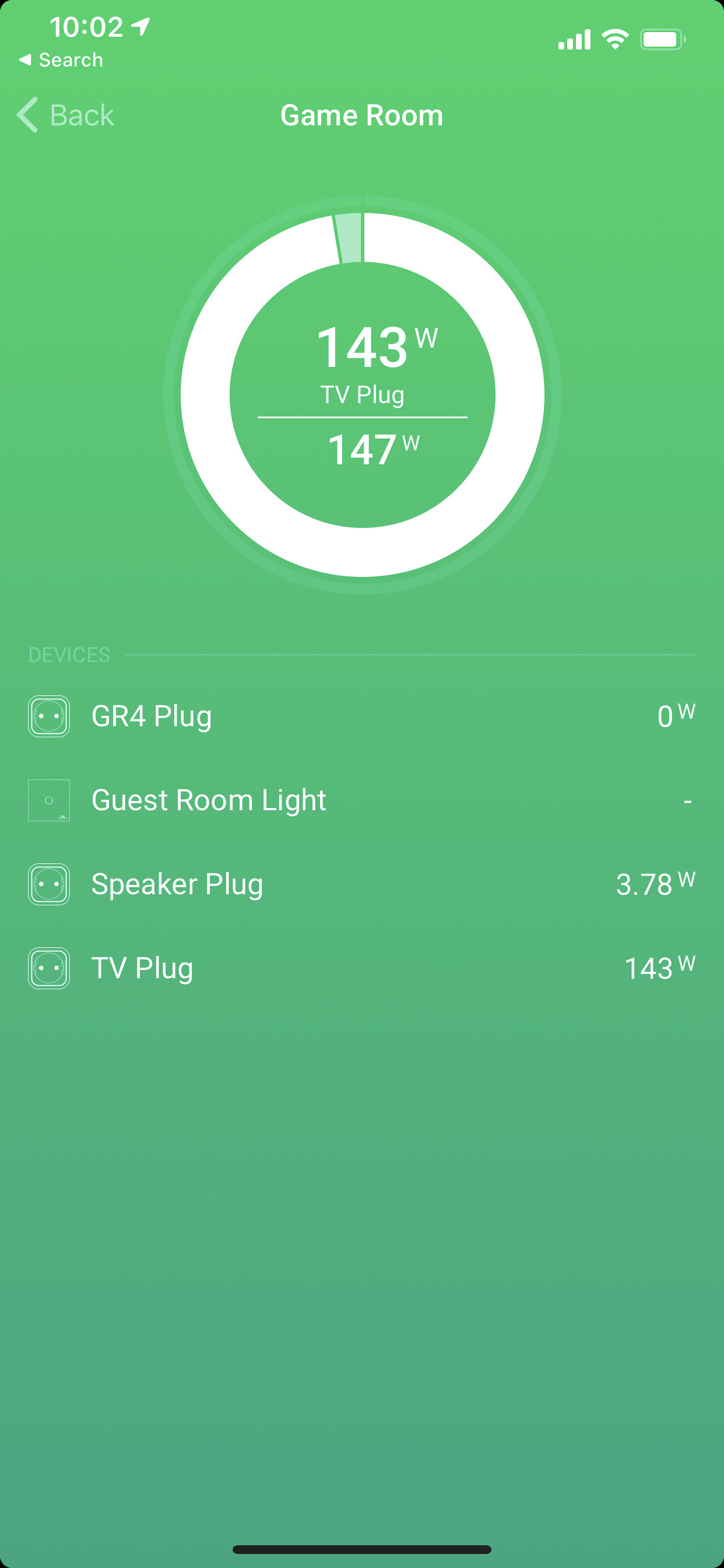Screenshot of a power consumption monitoring interface against a green ombre background. The interface is titled "Game Room" at the top. Below the title, a prominent white circle displays power usage information, indicating 143 out of a possible 147 watts for the TV plug in the center. Underneath, a list labeled "Devices" features icons for each connected electrical outlet. The first item, “GR4 Plug,” shows 0 watts. The “Guest Room Light” is grayed out with no power reading. The “Speaker Plug” shows 3.78 watts, and the “TV Plug” confirms 143 watts. Icons for an iPhone and the time, 10:02, are displayed at the top right corner.